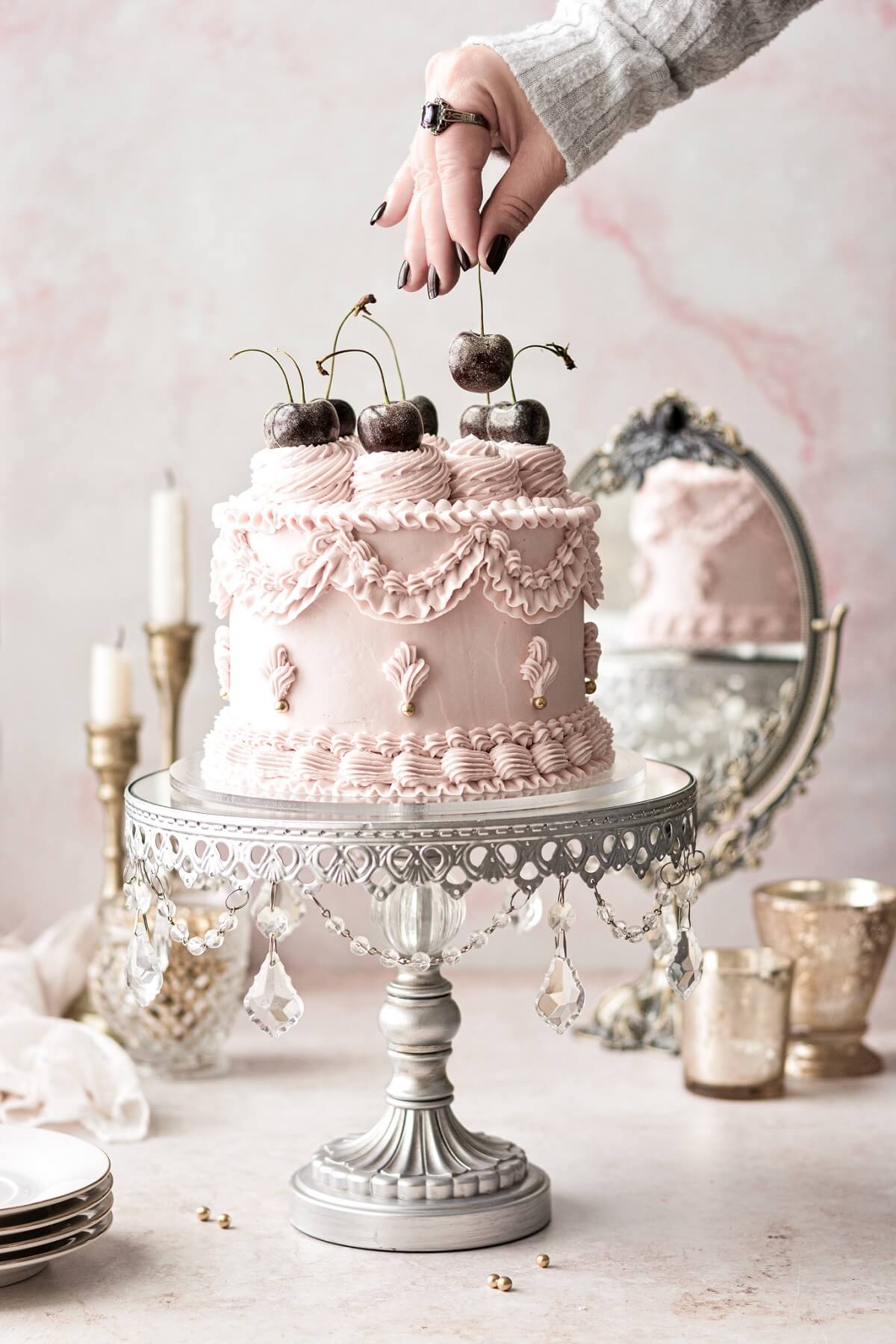This photograph captures a visually striking modern cake, which is the central focus of the image. The tall, pink cake is adorned with dark purple cherries that match the woman's fingernail polish. The cherries rest delicately on top of the cake as a woman's hand, adorned with a ring and with dark purple nail polish, reaches to pick one up. She is wearing a gray sweater.

The cake sits majestically on a silver pedestal, adding a touch of elegance, while the pedestal itself is embellished with linked gems hanging off its edge. The setting includes a white marble table, enhancing the sophisticated ambiance. Surrounding the cake are various elements that add to the tableau: to the left of the pedestal are plates and two candles, and to the right are two cups. A mirror in the background reflects part of the scene, creating depth. Scattered beads and fallen decorations add a whimsical touch to the composition, and the background is awash with a soft pink hue, complementing the cake. The overall scene exudes a sense of refined celebration.